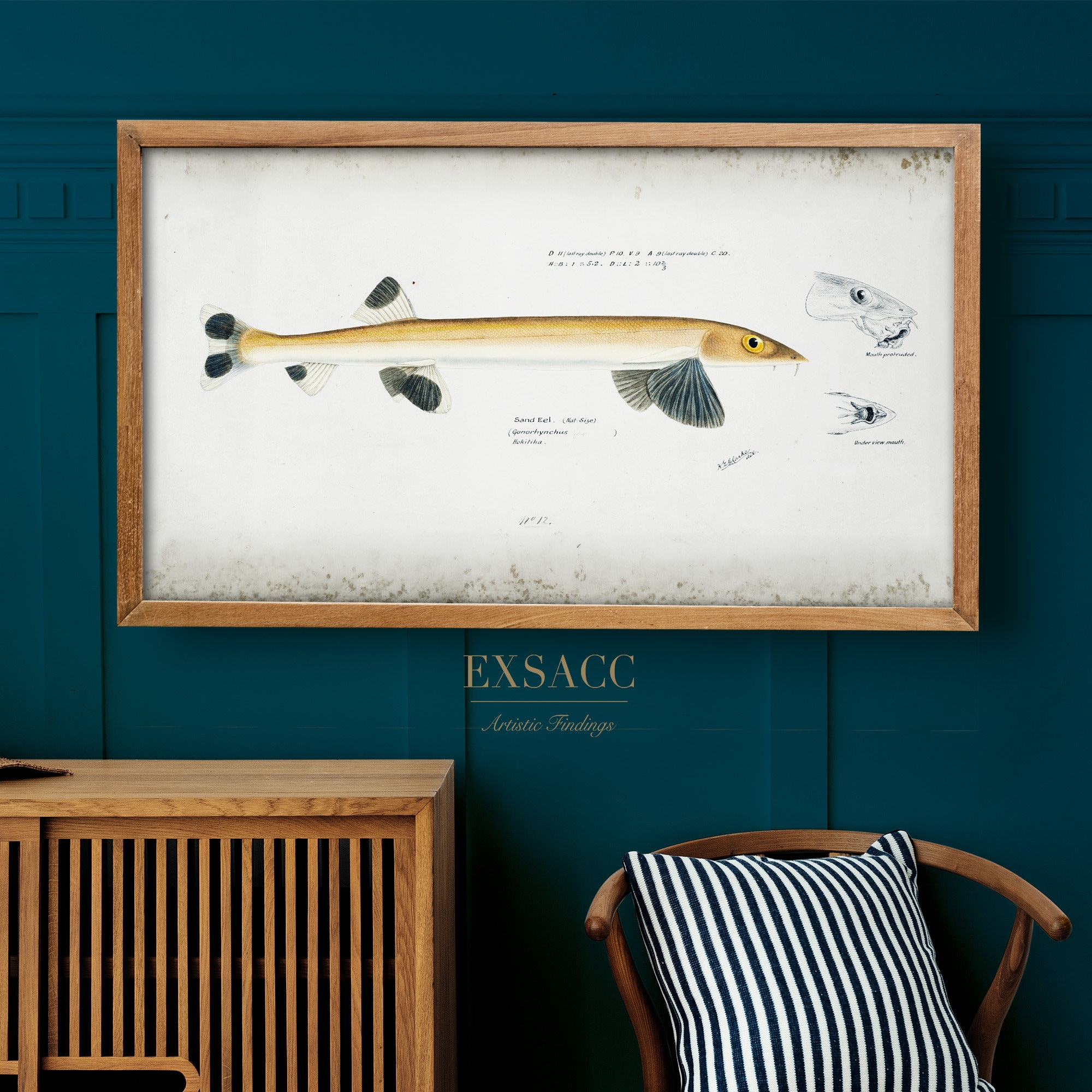The image depicts a cozy interior scene, possibly from a room, home, or shop. In the bottom right corner, there's a wooden chair adorned with a black and white striped throw pillow. The chair's backrest is partially visible, offering a glimpse of its structure. To the left of the chair stands a wooden cabinet or dresser featuring a distinctive design characterized by parallel vertical cut-out lines.

Above this piece of furniture is the focal point of the image: a framed artwork showcasing a long fish with brown and white coloration, accented by black spots and black fins. The fish stands out against a pristine white background, framed elegantly in wood. Completing the setting, the wall behind all these elements is painted a rich, dark teal, adding depth and warmth to the scene.